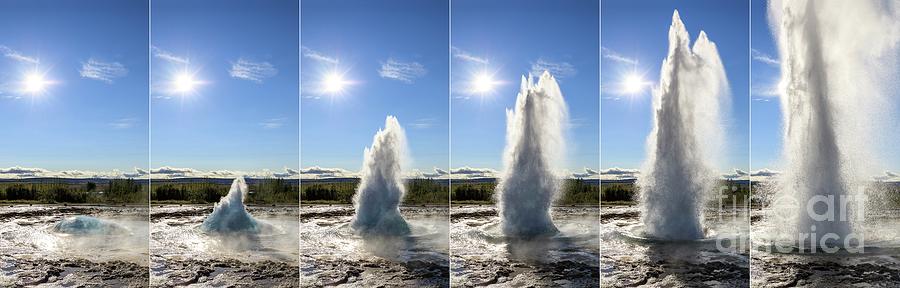The image is composed of six panels, each separated by a white line, capturing a sequence of a geyser erupting under a bright blue sky with soft linear clouds and a radiant sun. The leftmost panel shows the geyser as a small hole in the ground with minimal activity. Progressing to the right, the second panel has water beginning to rise from the ground. By the third panel, the eruption is clearly recognizable as a geyser, with water shooting up about three feet into the air. In the fourth panel, the geyser's water reaches around five to six feet. The fifth panel depicts the geyser surging to seven or eight feet, and in the final, rightmost panel, the geyser has erupted to an impressive height, extending beyond the top of the panel and spraying outward. A watermark reading "fine art america" in lowercase letters, with "fine" in a thinner font and "art america" in a bolder font, overlaps the fifth and sixth panels, marking the image.